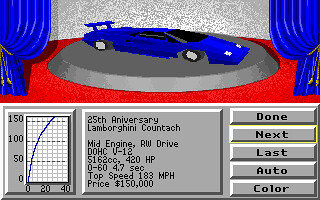This is a small, horizontal screenshot of a pixelated drawing depicting a Lamborghini car. The drawing appears to be a part of design software, showcasing the Lamborghini on a gray disc within a showroom setting. The car itself is characterized by white headlights, detailed white rims, a prominent spoiler, and blackout windows, standing out on a red floor. Enhancing the theatrical ambiance, there are blue curtains with gold ties framing either side of the vehicle.

Beneath the car image, there are several pieces of data embedded in the photo. On the left side, a graph is displayed, marked with vertical values of 150, 100, 50, and 0, while the horizontal axis indicates values of 0, 20, and 40. The graph's curve dramatically spikes from 0 to roughly 30. Centered on the bottom, there is a text box providing detailed specifications about the car, reading: "25th Anniversary Lamborghini Countach, Mid-Engine, RW Drive, DOHC V12, 5162 CC, 420 Horsepower, 0 to 60 in 4.7 seconds, Top Speed 183 mph, Price $150,000." On the right side of the screenshot, five vertically aligned buttons are labeled in black letters as follows: Done, Next, Last, Auto, and Color.